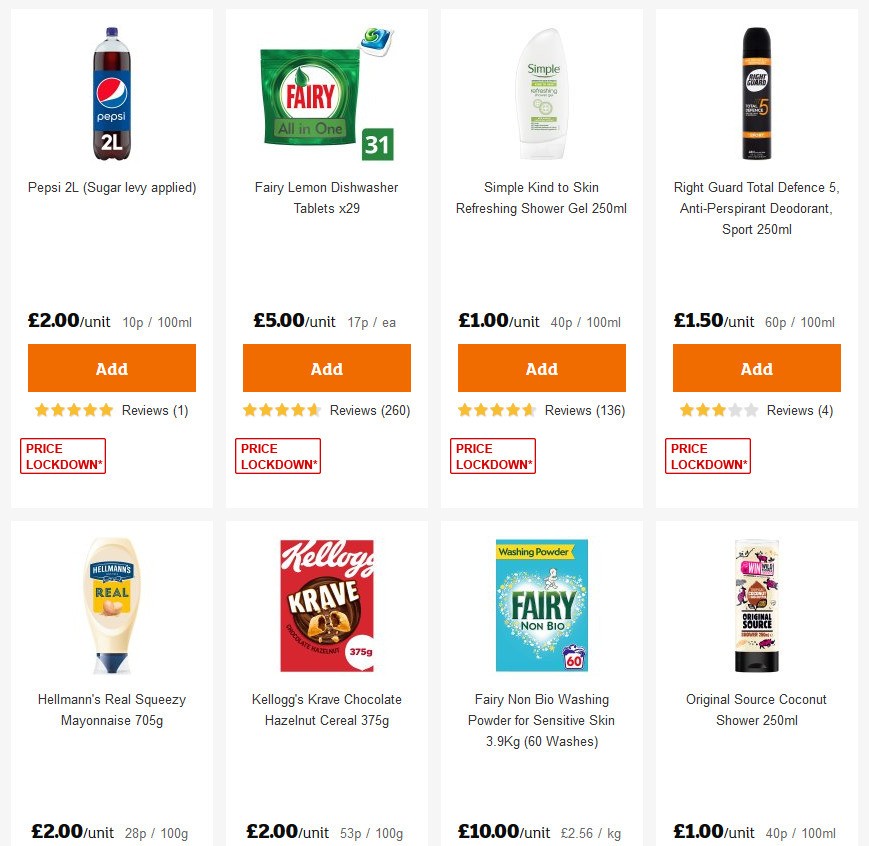Screenshot of an Online Shopping Page:

The screenshot captures an online shopping page with a clean, white background. The page is organized into a grid format with 8 product listings, arranged in two rows with four items each. Each product is presented within a distinct rectangle segment.

**First Row:**
1. **Pepsi Soda (2 liter)**
   - Price: £2 per unit
   - Button: Orange with white text reading "ADD"

2. **Fairy Lemon Dishwasher Tablets (29 count)**
   - Price: £5 per unit
   - Button: Orange with white text reading "ADD"

3. **Simple Kind to Skin Refreshing Shower Gel (250 milliliters)**
   - Price: £1 per unit
   - Button: Orange with white text reading "ADD"

4. **Right Guard Total Defense 5 Antiperspirant Deodorant Sport (250 milliliters)**
   - Price: £1.50 per unit
   - Button: Orange with white text reading "ADD"

**Second Row:**
1. **Hellmann's Real Squeezy Mayonnaise (705 grams)**
   - Price: £2 per unit
   - Button: Orange with white text reading "ADD"

2. **Kellogg's Krave Chocolate Hazelnut Cereal (375 grams)**
   - Price: £2 per unit
   - Button: Orange with white text reading "ADD"

3. **Fairy Non-Bio Washing Powder for Sensitive Skin (3.9 kilograms, 60 washes)**
   - Price: £10 per unit
   - Button: Orange with white text reading "ADD"

4. **Original Source Coconut Shower Gel (250 milliliters)**
   - Price: £1 per unit
   - Button: Orange with white text reading "ADD"

Each listing includes an orange "ADD" button with white text positioned directly underneath the product details, allowing customers to easily add items to their cart.